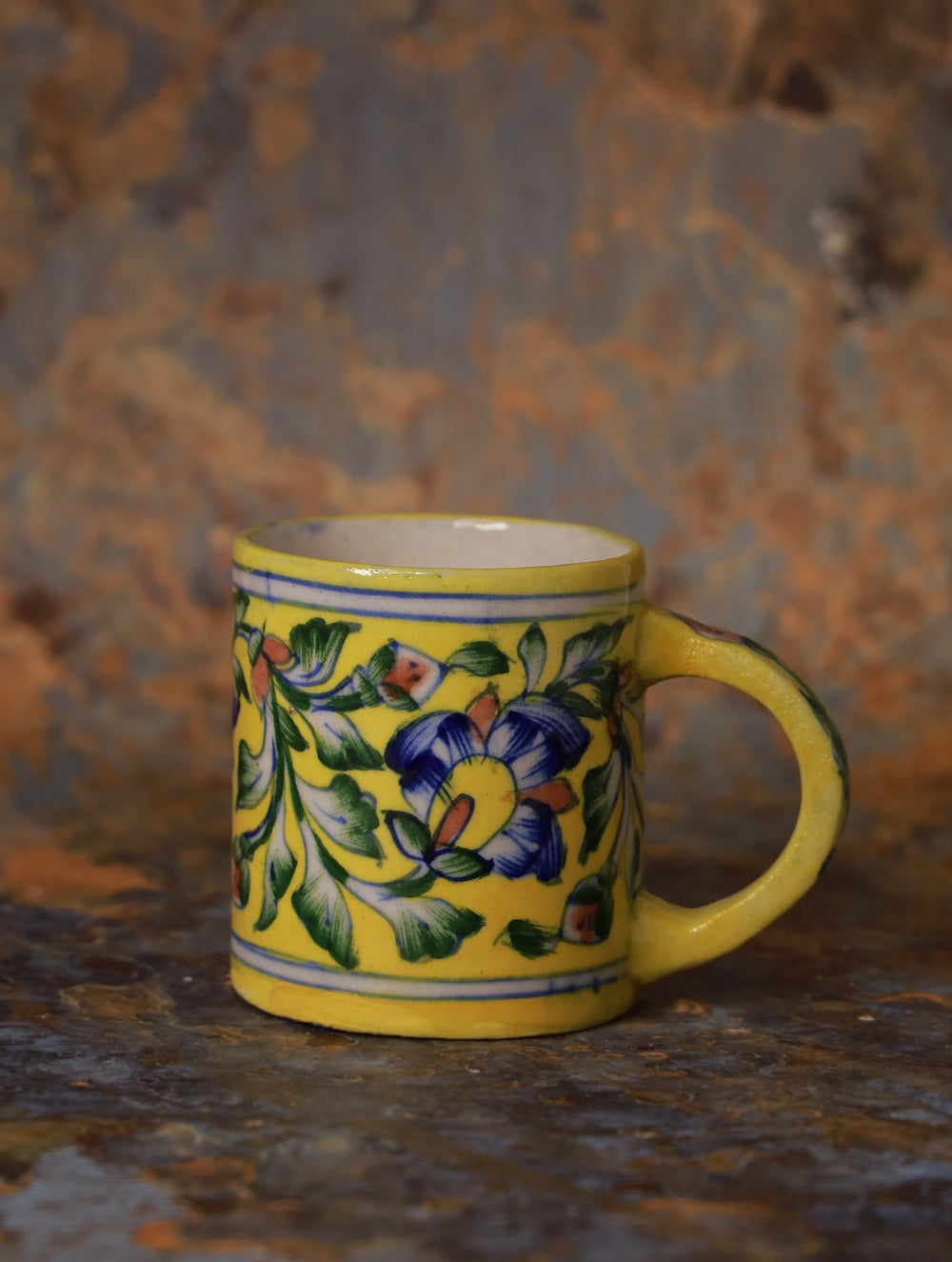The image depicts a hand-decorated coffee mug with a yellow background, adorned with botanical designs featuring blue and red flowers accented with green leaves. The mug's exterior includes white sections bordered by two sets of blue lines—one near the rim and another near the base. The mug's interior is white, and its yellow handle, positioned on the right side, adds to its intricate design. The setting includes a weathered, rust-streaked gray surface both beneath the mug and in the backdrop, giving the impression of an aged, industrial environment. This contrast draws attention to the vivid and thoughtfully crafted details of the mug itself.